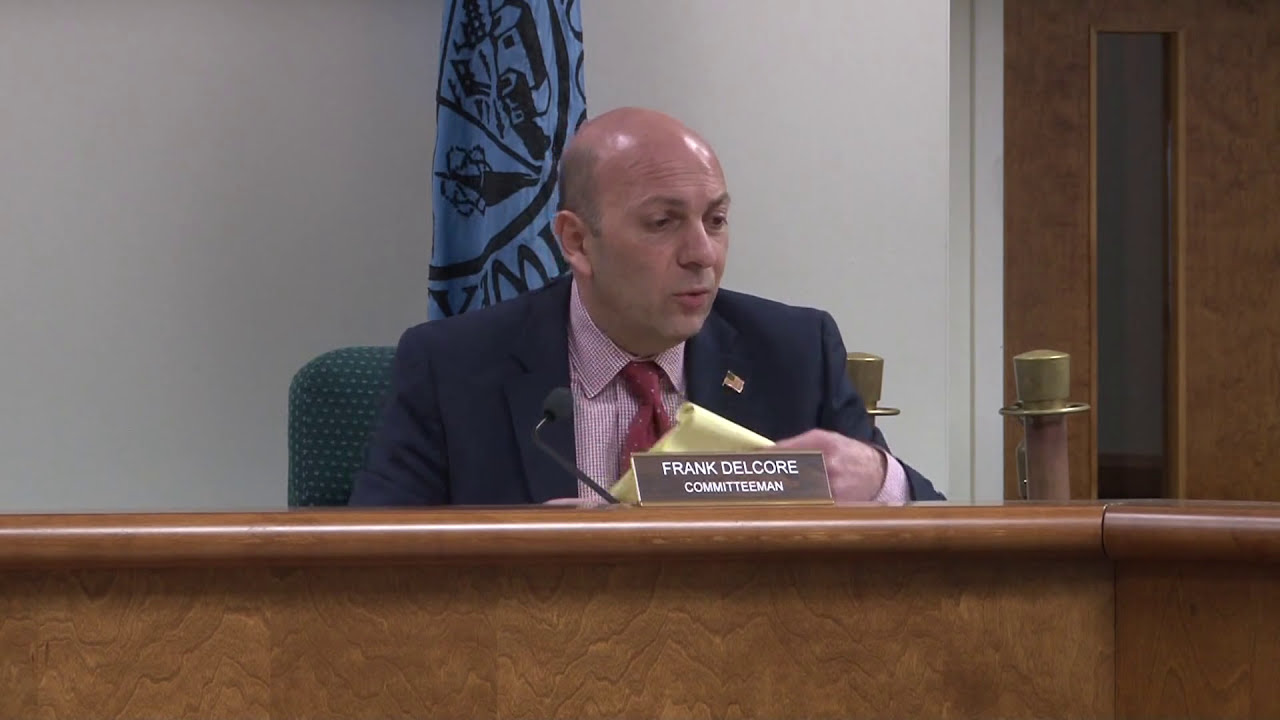In the photograph, an older, bald man sits behind a large, shiny brown wooden desk. His head is notably shiny and he is discernibly Caucasian. Dressed in a navy blue suit, he sports a pink shirt adorned with a reddish tie that has white dots, and a U.S. flag pin on his left lapel. The man is seated in a green chair dotted with white spots. Directly in front of him, mounted on the desk, is a brown placard with white capital letters that read "Frank DELCORE" and "COMMITTEE MAN" below it. To his right, there is a brown wooden door with a rectangular window. The backdrop features white walls, a couple of poles creating a barrier behind him, and a blue and black flag, whose details are indiscernible from this view. Additionally, there is a black speaker angled towards him on the left.